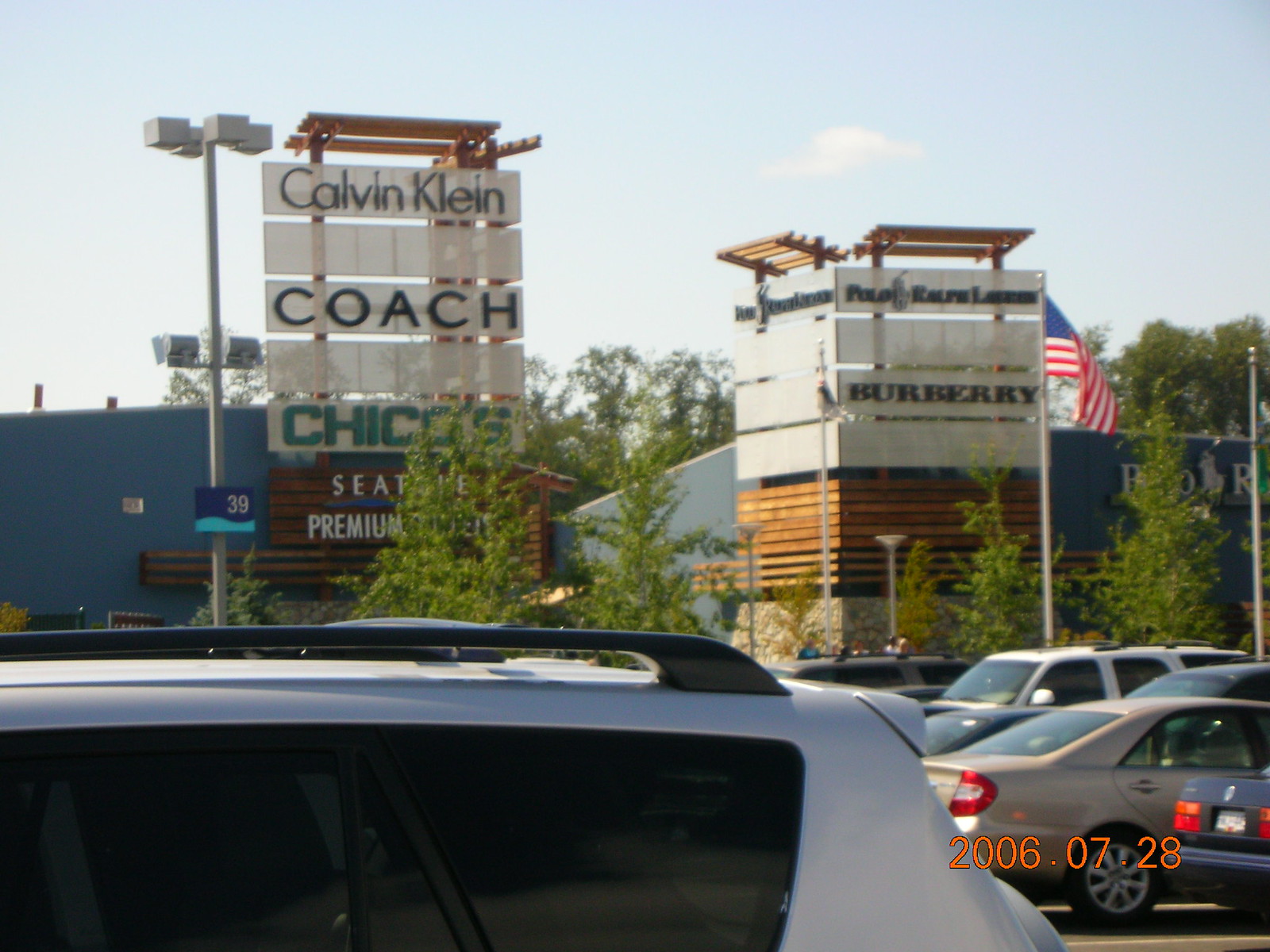The image depicts a bustling premium outlet mall in Seattle, with a clear view of the parking lot taken from ground level. The contemporary architecture of the outlets features sleek blue buildings adorned with wooden accents above the store signs, adding a touch of rustic elegance. Prominently displayed store signage includes well-known brands like Calvin Klein, Coach, Chico's, Burberry, and Polo Ralph Lauren. An American flag flutters proudly in front of the outlets, enhancing the patriotic ambiance of the scene. The parking lot is filled with a variety of vehicles in diverse colors, such as white, tan, and black, indicating that the mall is a popular shopping destination. In the background, partially obscured by a tree, the word "Seattle" is visible, confirming the location.